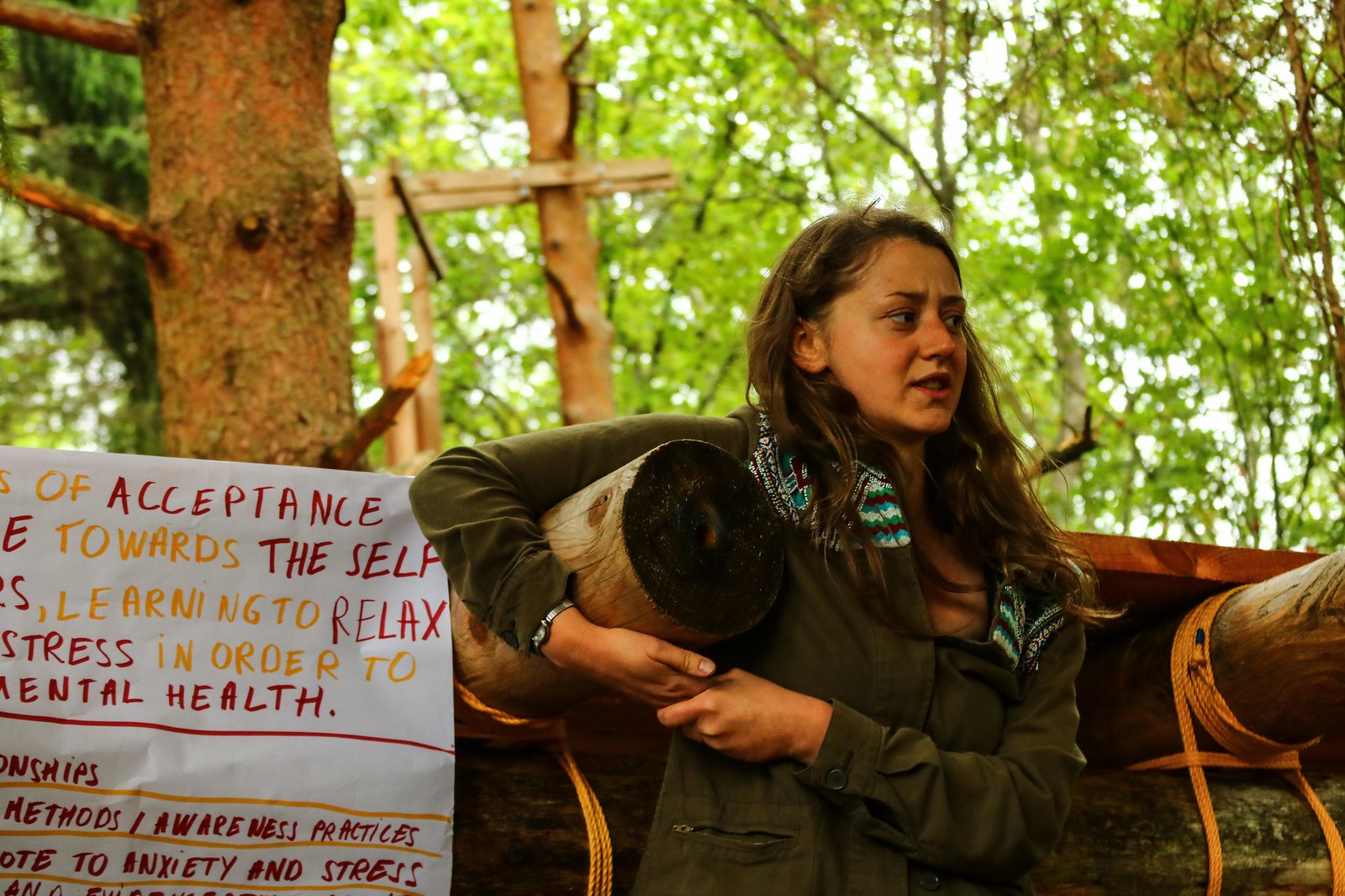The photograph depicts a woman, approximately in her 20s or 30s, with long brown hair and fair skin, wearing an olive green jacket layered over a light-colored lapel top. She is leaning against a log, which appears to support a wooden platform behind her, using her right arm to wrap around it. The platform is secured with sisal-type rope and flanked by another similar log. She gazes off to the right of the frame. In the bottom left corner of the image, there's a partially visible white sign with yellow and red text that includes fragments of sentences about self-acceptance, learning to relax, and methods or awareness practices for anxiety and stress. The background features a dense array of trees, suggesting an outdoor retreat setting in the woods.